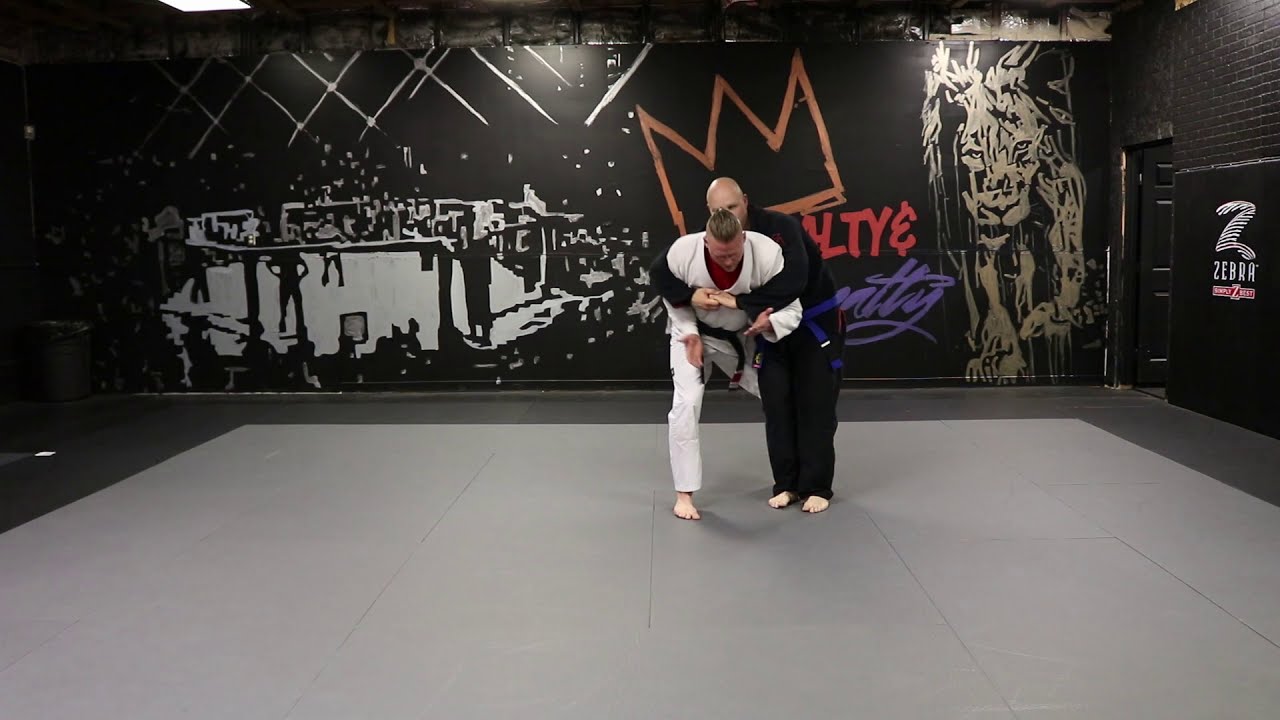In a studio gym with gray mat flooring and black brick walls, two men are practicing martial arts, possibly taekwondo or karate. The studio features a large black mural with the image of a fighting ring, a lion, and an orange crown, prominently showcasing a logo ending in 'LTY' or 'TTY'. On the mat, a bald man in a black gi with a blue belt is gripping another man from behind. This second man, who has a distinctive wide mohawk of brown hair, is dressed in a white gi with a black belt. The man in the white gi is hunched over and appears to be demonstrating or attempting a counter-move, his hand lifted in a defensive position.